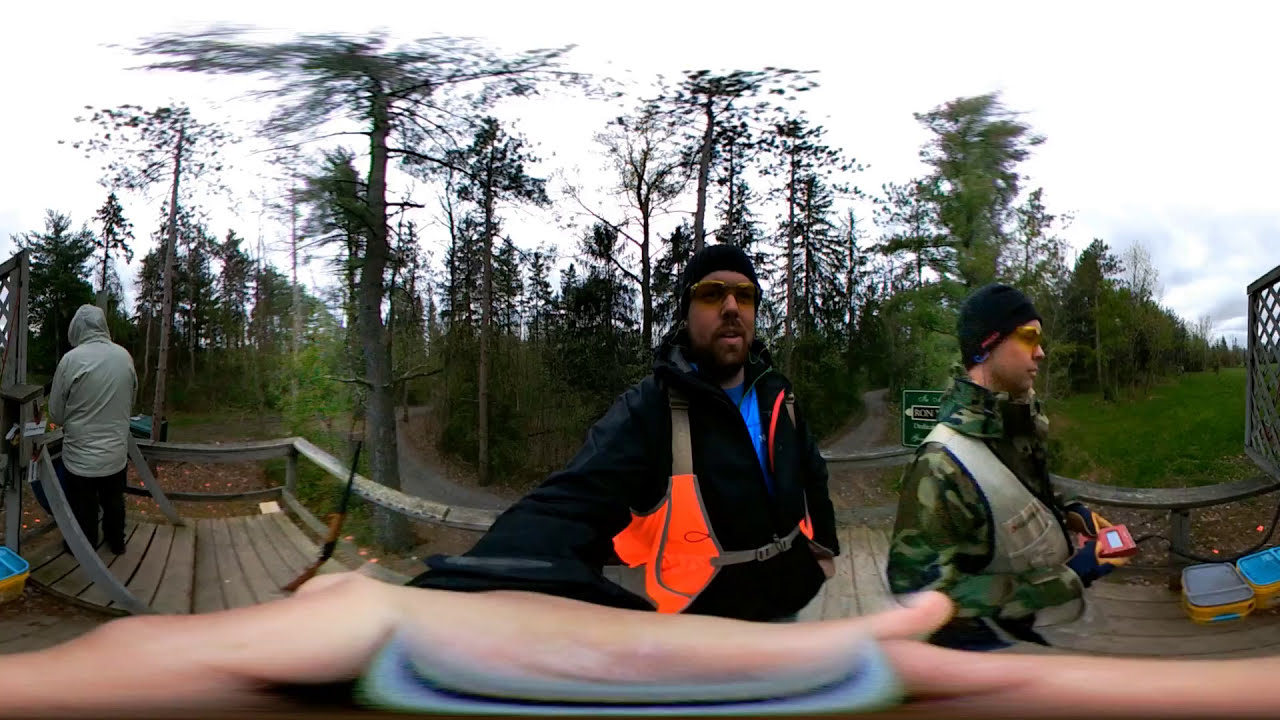An outdoor photograph captures a picturesque moment of three men casually hanging out on a wooden deck set against a natural backdrop. This deck appears to overlook a forested area with light and dark green trees and a cloudy sky. At the center of the image, a man with a full beard and mustache is standing, wearing a black jacket with a neon orange trim, a blue undershirt, a black knit ski cap, and sunglasses, making him the focal point. To his right, there is a younger, clean-shaven man in a camouflage jacket with a beige vest, black rimmed glasses, and a black beanie, who is holding a red controller in his hands. On the far left, standing with his back to the camera and looking towards the left side of the image, is a person in a hooded silver (or beige) jacket and dark pants, possibly jeans. The deck surface is a consistent gray color that matches the road in the background. The entire bottom fourth of the image is dominated by this deck, while the middle right section features the green grass of an open field. On the far left, beyond the deck, different colored trees and a couple of roads can be seen. The group appears to be enjoying a serene moment in nature, perhaps on a camping trip or outdoor excursion.